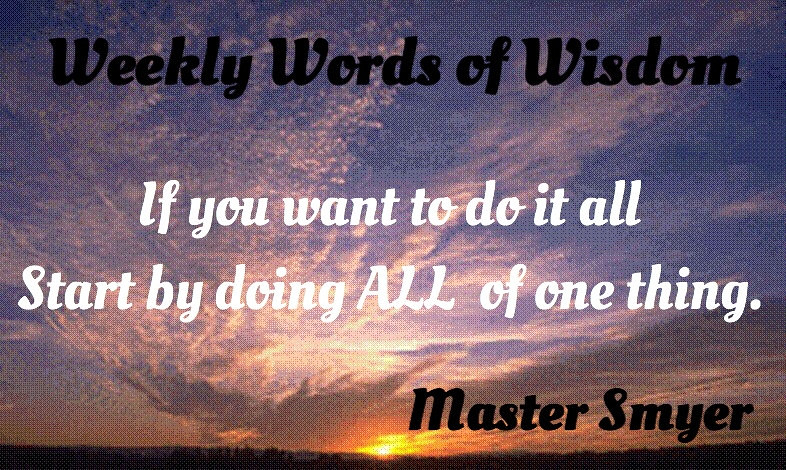The image is a vibrant and colorful photograph of a sunset, commonly used for inspirational messages or memes. The sun is nearly at the horizon, casting a brilliant orange glow that blends into shades of pink, purple, and blue across the sky. Thin clouds are spread across the expanse, some dark near the horizon and others lit up in pink hues higher up. At the very bottom of the image, you can see some trees. 

Across the top in black text, it reads, "Weekly Words of Wisdom." Below this, in white text, it says, "If you want to do it all, start by doing ALL of one thing," with the word "ALL" in capital letters. At the bottom, in black text again, it credits the quote to "Master Smyer, S-M-Y-E-R." The overall effect is a serene yet motivational scene designed to inspire.